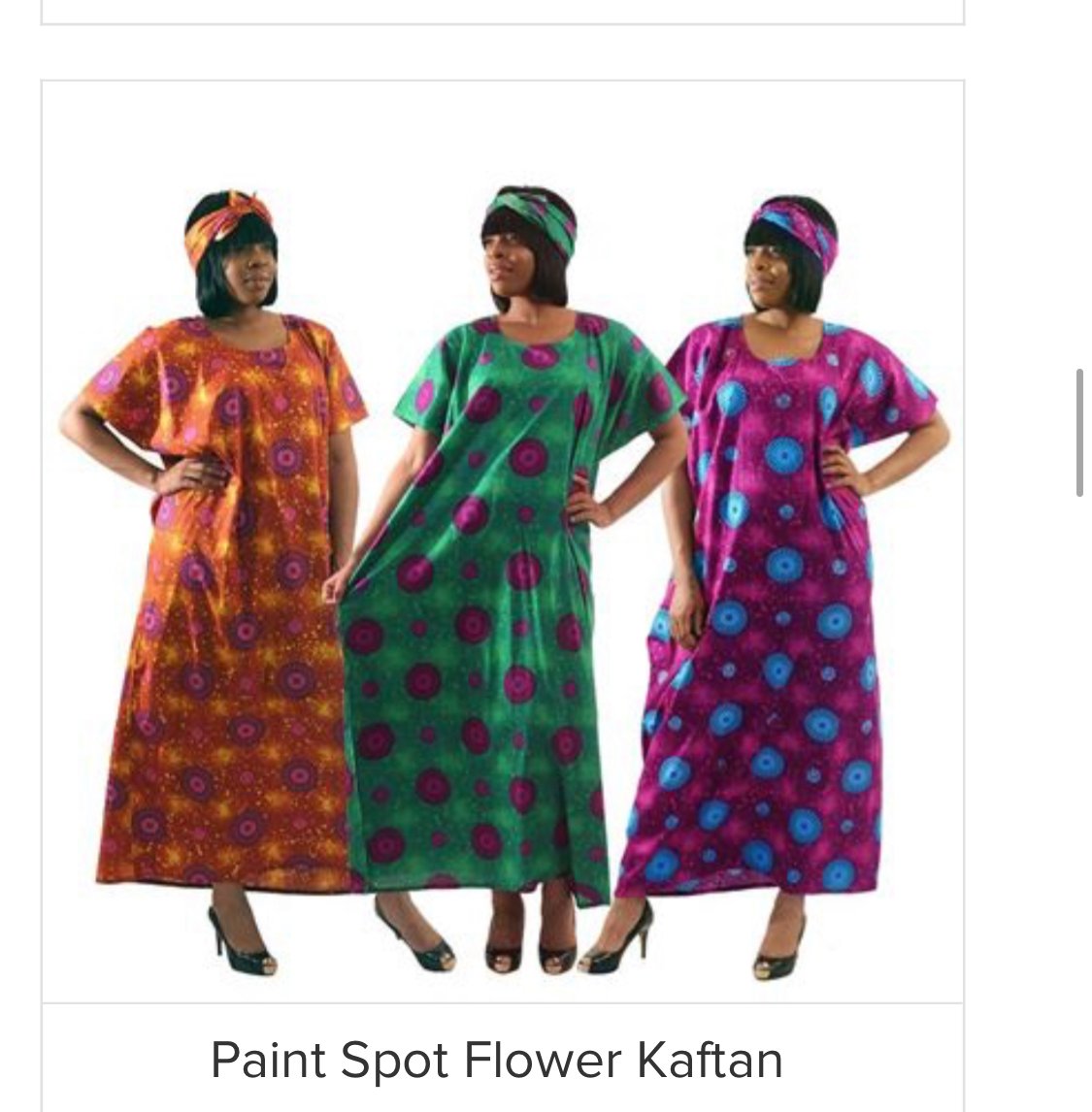The image features a black woman positioned side-by-side in three different colored kaftans, each with the same floral pattern but in various color schemes. On the far left, she is depicted in an orange, purple, and pink kaftan; the middle shows her in a green kaftan adorned with pink circles; and on the far right, she is in a purple kaftan with blue circles. In each instance, the woman, who has chin-length black hair with a straight bang and wears a matching headband or scarf, stands with one hand on her hip. Her footwear consists of black peep-toe high heels. Text at the bottom of the image reads "Paint Spot Flower Caftan" in black. The photo has a very thin gray pinstripe border and a white or translucent background, giving it a digitally edited appearance.